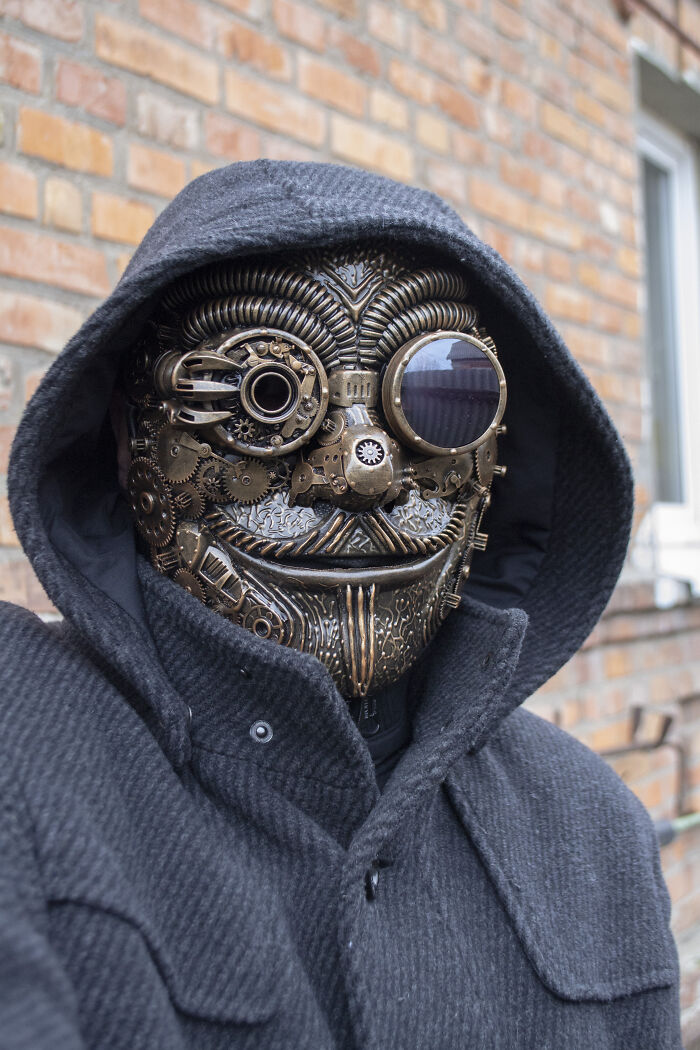The photograph depicts a figure, possibly a man or a woman, dressed in a blue wool hooded jacket, leaning against a red brick wall with a white window sill to the right. The person wears a steampunk-inspired mechanical mask crafted from copper and silver materials, featuring detailed and intricate parts. The mask exhibits a slightly smiling mouth, a nose with a gear at its tip, and eyebrows made of bent springs. The left eye of the mask is designed to look like a glass lens outlined in copper, with three claws gripping its exterior, marked by a black slit. The other eye resembles a mirrored goggle. The cheeks are adorned with gears, and a mechanical mustache adds to the mask's complexity. The figure looks directly at the camera, creating a slightly eerie yet intriguing impression, further enhanced by the outdoor lighting.